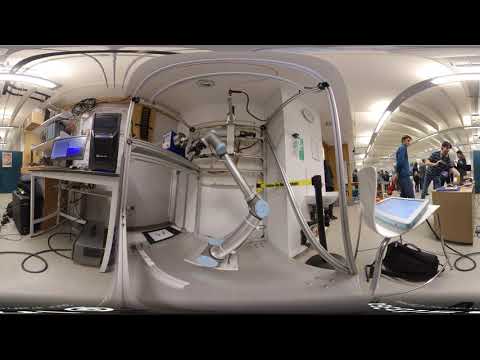The image is a panoramic view of a high-tech research lab that appears well-lit and spacious. At the center, a large robotic arm is enclosed in a white, panel-surrounded area, reminiscent of a space station module. To the left, a computer on a tall table is accompanied by a tower desktop, highlighting the heavy presence of technology in the lab. To the right, a white chair with a computer screen and bags underneath it sits next to a work pad, suggesting an organized setup for detailed tasks. The floor is adorned with various wiring, consistent with the lab's technical environment. In the background, on the right-hand side, a group of people—possibly researchers or doctors—stand observing. The room itself is white and has an underground feel, exuding a sterile and controlled ambiance.